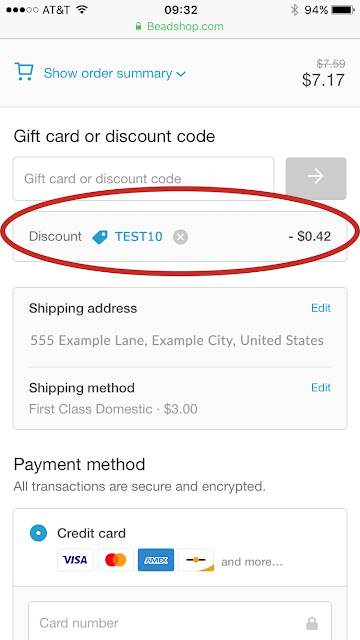A detailed screenshot shows a smartphone displaying a webpage from beadshop.com, with the cellular carrier AT&T visible at the top. The current time reads 9:32, and the battery level is at 94% while connected via Bluetooth. The webpage features a blue shopping cart icon and a "Show order summary" button. To the right of this, the subtotal is listed as $7.17. Below this section is a field for entering a gift card or discount code, with a red oval highlighting the word "discount" next to a price tag noting "test 10" for a discount of minus 42 cents. 

Further down, the shipping address is displayed as "555 Example Lane, Example City, United States," with an "Edit" option above it. The shipping method is specified as "First Class Domestic" costing $3, with another "Edit" option to the right. Under "Payment Method," it assures that "All transactions are secure and encrypted." Various payment icons are shown, including those for Visa, MasterCard, Amex, and Discover, followed by a card number field accompanied by a lock icon for security.